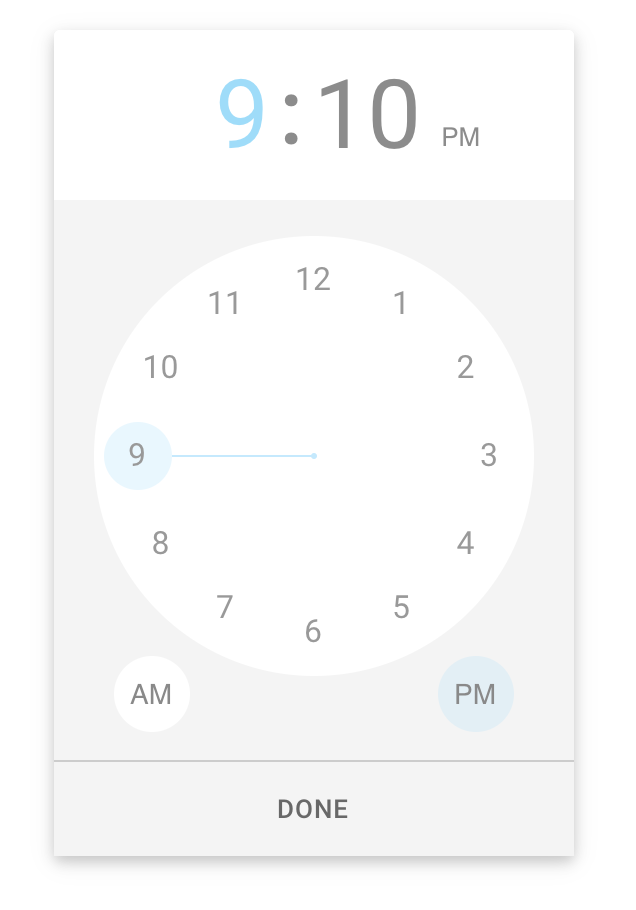The image depicts a clock application interface. The top section features a light blue "9" followed by a gray "10" and a small "p.m.", indicating the time is 9:10 PM. Below the time, a clock face is displayed with numbers 1 through 12 in a circular arrangement. On the left side of the clock, it says "AM" while on the right side, it says "PM". A shadow effect is visible on the left, right, and bottom edges of the interface. At the bottom of the image, we see the word "done," likely a button for confirming the time.

In the center of the clock face, a bar extends to the left, pointing to a grayish circle around the number 9. The bottom-right side of the clock has another grayish circle. The main display circle in the center is white, set against a gray background, with the top section being white. The entire setup suggests a user interface design for setting and displaying time within a clock application.